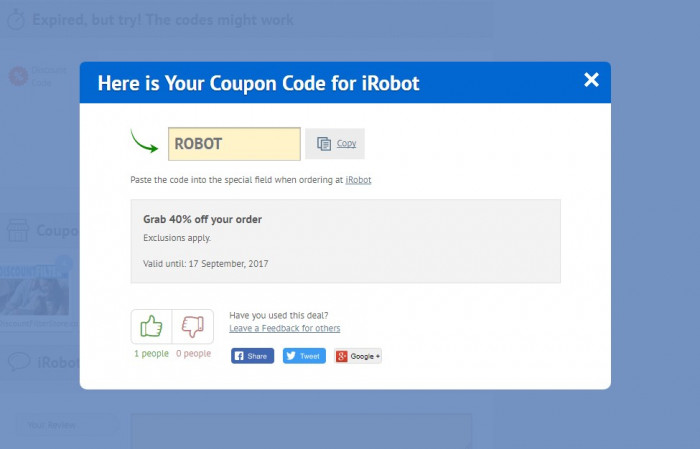In the foreground, there is a pop-up window offering a coupon code for iRobot. The pop-up is set against a background where it appears someone was initially searching for a coupon code. Dominating the center of the pop-up is a blue rectangle displaying the message "Here's your coupon code for iRobot" in white text. In the top right corner, there's a white "X" icon for closing the window.

Adjacent to the main message, a green arrow pointing to the right directs attention to a text box containing the coupon code: "ROBOT." Next to this text box, there are two pieces of paper icon enclosed in a gray box with the word "Copy" underlined, indicating that you can click to copy the code.

Below the main section, instructions in regular text advise users to paste the code into a special field when ordering at iRobot to receive 40% off, though exclusions apply. This offer is valid until September 17, 2017. The offer details "Grab 40% off your order" are highlighted in bold and placed within a large gray rectangle.

At the bottom of the pop-up, there are options for feedback: a green thumbs-up icon and a red thumbs-down icon, both in gray boxes. So far, one person has given a thumbs-up, and no one has given a thumbs-down. There is also a prompt encouraging users to "Leave feedback for others," which includes a link. Additionally, there are social media sharing options for Facebook, Twitter (represented with the icon of formerly known Twitter as X), and Google+.